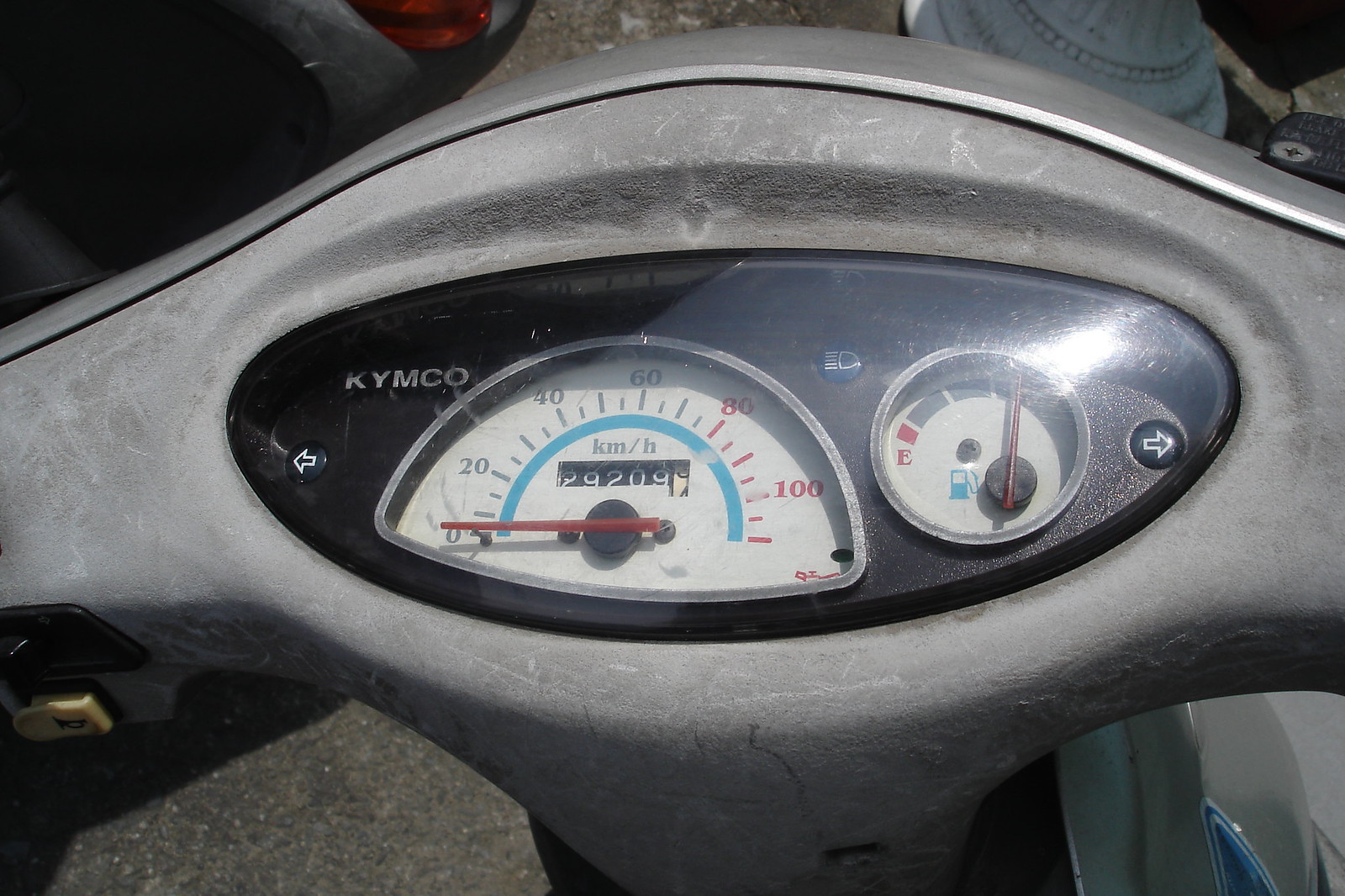This detailed photograph captures the top view of a KYMCO motorcycle's gauge cluster set against an outdoor backdrop. Showcasing a comprehensive and organized layout, the gauge cluster prominently features the silver "KYMCO" branding in the upper left corner. Right below it is a left turn indicator arrow. Dominating the center is the speedometer, meticulously calibrated in kilometers per hour, ranging from 0 to 100 in 20 km/h increments and color-coded in white, red, and yellow. The odometer beneath the speedometer displays the mileage, reading at 29,209 kilometers. Adjacent to the speedometer, a fuel gauge mirrors the color scheme of white, blue, and yellow. Nestled beside the fuel gauge is a headlight symbol, providing essential information at a glance. To the extreme right, a right turn indicator arrow completes the cluster. The entire gauge cluster is set within a rectangular, gray-colored background, offering a sleek and cohesive aesthetic that compliments the motorcycle's practical functionality.